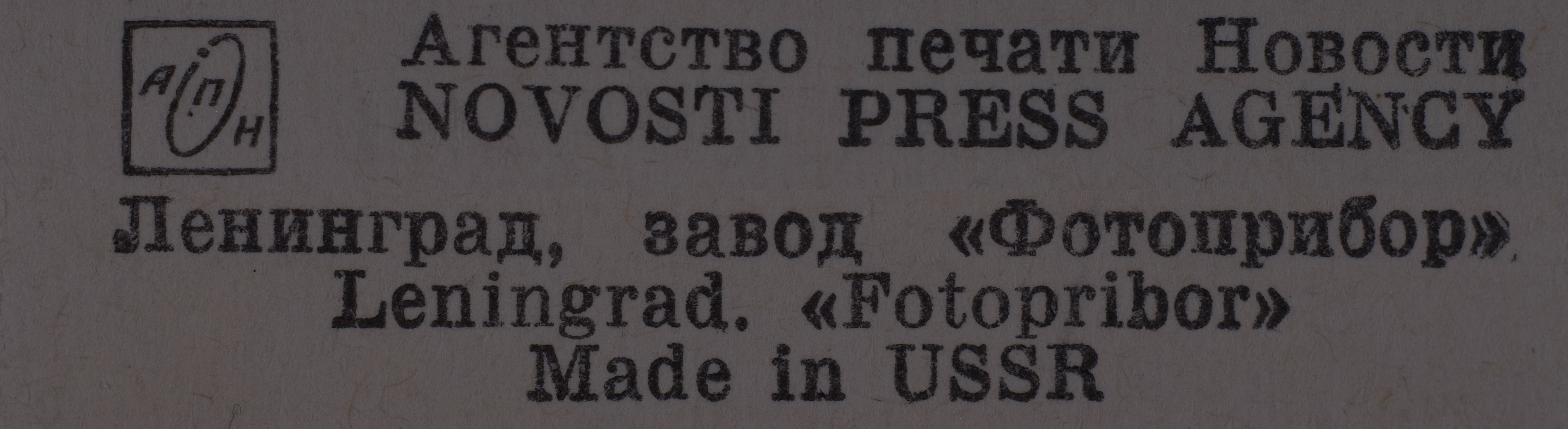This image showcases a rectangular-shaped sign with a dark gray background and black text. The sign prominently displays "Novosti Press Agency" in English, accompanied by Russian text above it. On the left side, there's a distinctive logo featuring the letters "A-N-H," with the "N" encircled within a box. The Russian text indicates the connection to Leningrad and contains another name that is difficult to decipher. Additionally, the sign confirms its origin with the words "Made in USSR," emphasizing its historical context and Soviet-era origin.